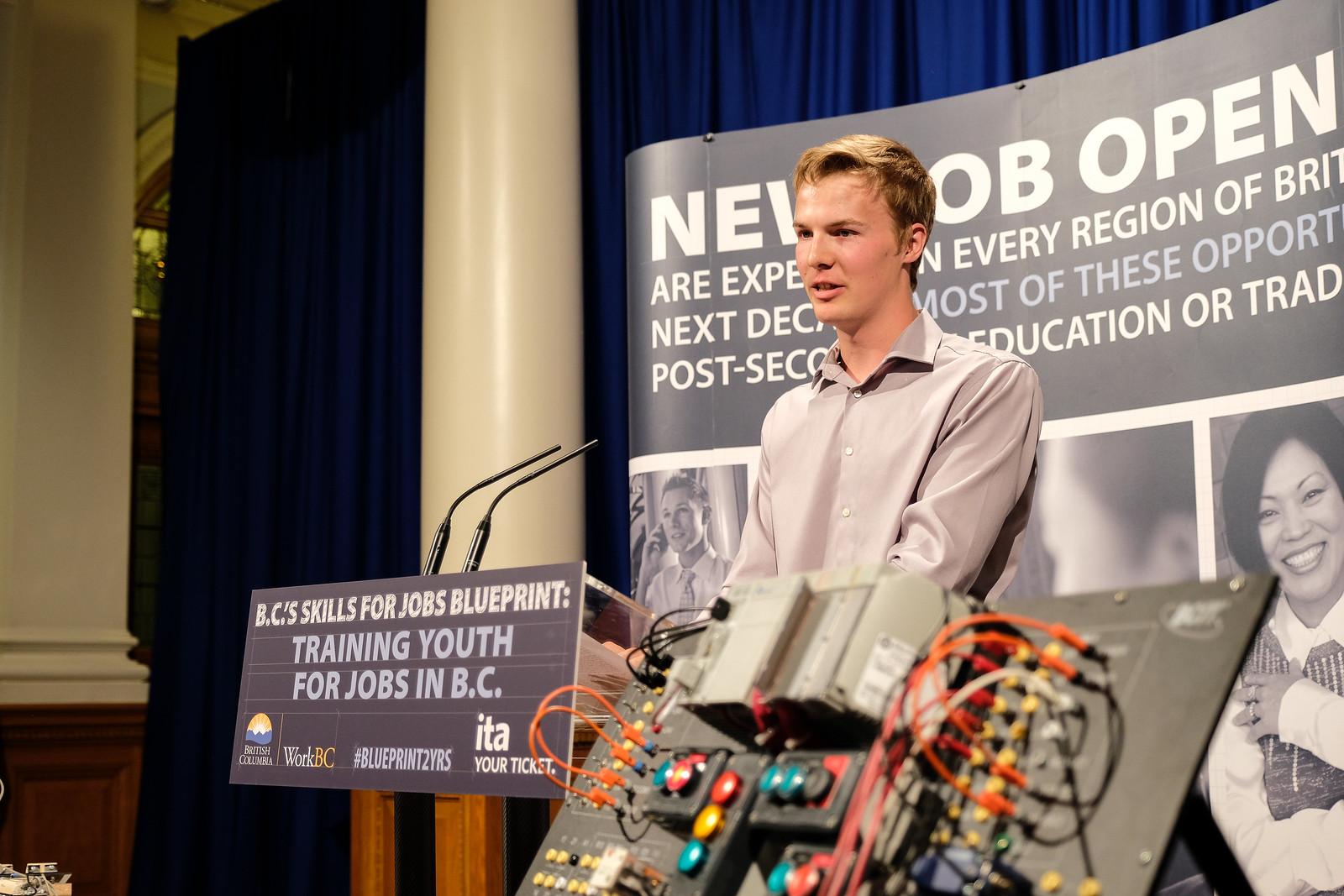The photograph captures an indoor event, likely a conference or speaking engagement, centered around youth job training in British Columbia. A young man with combed back blonde hair, wearing a gray long-sleeve shirt, stands behind a podium adorned with a blue banner reading "BC's Skills for Jobs Blueprint, Training Youth for Jobs in BC." The podium is equipped with two microphones. In front of him is an electronic device resembling a circuit board, detailed with red and yellow wires, and colored buttons, suggesting he might be discussing tech-related job opportunities. Behind him is a large poster featuring text and black-and-white images of smiling individuals, partially obscured but implying opportunities or new job openings. The background includes thick white columns and blue theater curtains, adding to the formal ambiance of the setting. Sponsors like Blueprinters, ITA, and Your Ticket are also acknowledged in the scene, further emphasizing the professional and educational nature of the event.